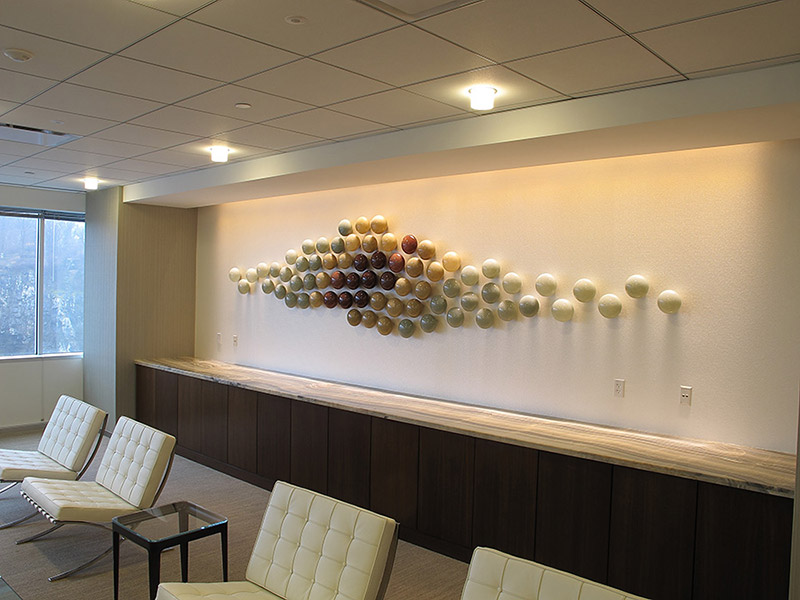The image depicts a stylish interior, likely part of a conference room, hotel, or similar gathering space. The room is viewed from a right angle, highlighting a modern aesthetic with four cushioned, armless chairs upholstered in white leather. These chairs are arranged around a sleek glass table with black legs. The backdrop is a striking feature wall painted white, showcasing an eye-catching art installation made up of various coloured orbs. These orbs progress in shades from white on the periphery to dark reddish-brown in the center, forming an amorphous, visually compelling design. Additional elements in the room include a recessed wall with built-in shelves, complete with closed wooden cupboards, and four electrical plugs. Overhead, three suspended lights illuminate the space. On the left side of the room, a window offers a view of trees or plants, while a carpet with an industrial pattern covers the floor.